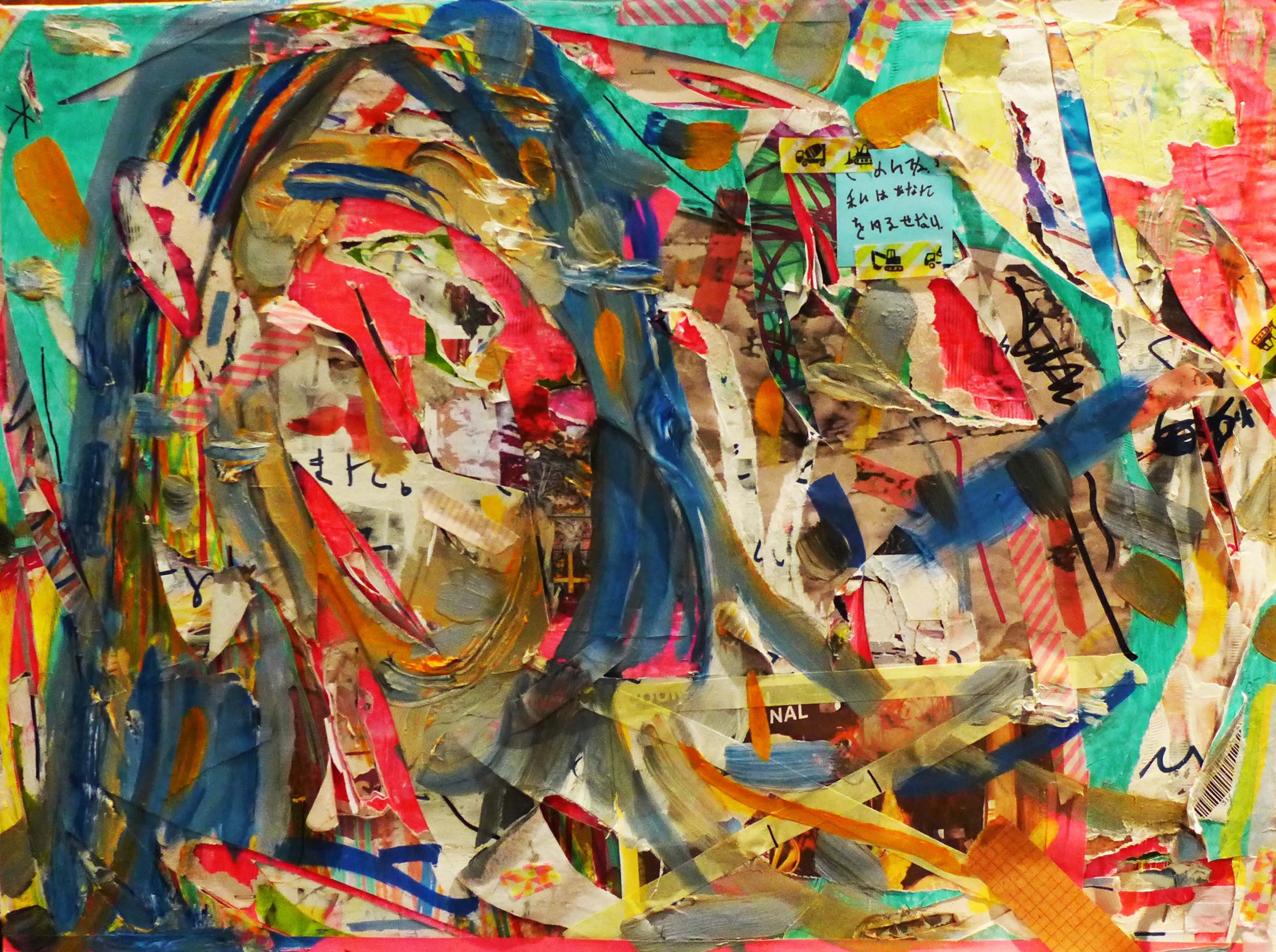This image depicts a chaotic and vibrant art piece, possibly an abstract or experimental project, featuring a combination of mixed media on a board. Dominated by an outline of a woman with blue hair, the artwork showcases a plethora of colors including blues, teals, reds, blacks, greens, and yellows. Various materials such as ripped paper, ribbon, pieces of tape, strings, and even what appears to be a receipt are glued haphazardly across the surface. A sticky note with non-English, possibly Asian, characters is prominently placed in the top right corner. Additional elements like a book cover and remnants of graffiti-like markings suggest a layered composition, evoking a sense of both clutter and creativity. The jumbled arrangement and diverse textures contribute to its abstract nature, creating an impression of spontaneity and emotional expression.